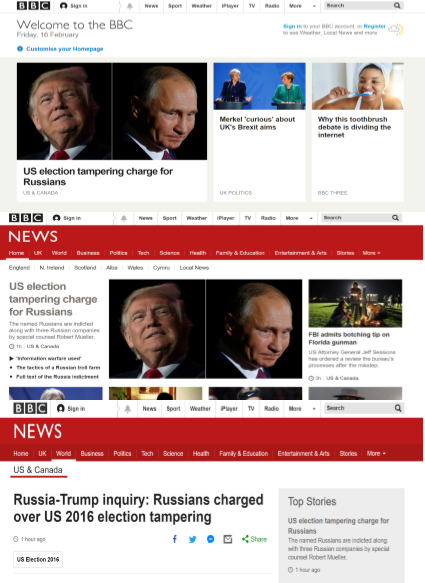Screenshot from the BBC Website:

The image is a screenshot from the BBC website, prominently displaying the iconic BBC logo composed of four cubes in the upper left-hand corner. The main navigation bar below the logo features options for News, Sports, Weather, iPlayer (partially obscured), TV, Radio, and More. On the upper-right corner, there is a search bar. "Welcome to the BBC" is seen as a header message.

The main content of the page has a headline reading "U.S. election tampering charge for Russians," accompanied by a photo of Vladimir Putin to the left and Donald Trump to the right. Below this headline, there is another news highlight about a debate on stage titled "Merkel curious about UK Brexit," featuring an image of Angela Merkel alongside an unidentified individual.

Further down, an article with a peculiar image of a woman brushing her teeth discusses "Why this toothbrush debate is dividing the internet."

The screenshot seems to reveal multiple layers or sections of the website, each reiterating similar news themes. As the viewer scrolls down, the header changes to red with the word "News" prominently displayed. The repeated article about U.S. election tampering charges features the same photograph of Trump and Putin, with additional photos underneath and a headline to the right about the FBI admitting to botching a tip on a Florida gunman.

At the bottom of the screenshot, the page header changes to "U.S. & Canada," presenting the same news about Russian interference in the 2016 U.S. election but without photos.

Overall, the screenshot appears to juxtapose three different sections or versions of the BBC website, cohesively summarizing the major news themes across different regions or page layouts.